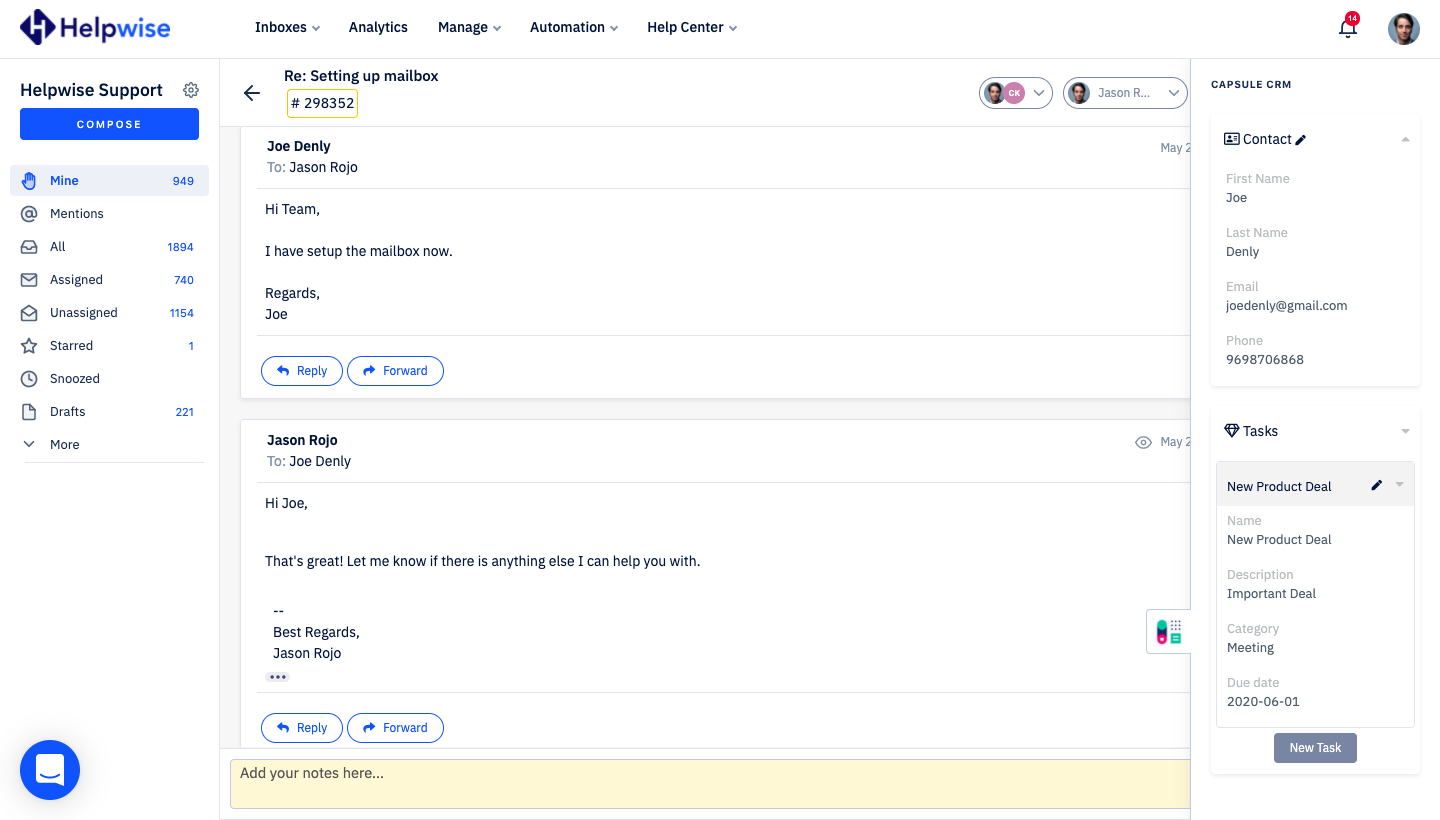The image is a screenshot of a web page with a white background. In the upper-left corner, the name of the company, HelpWise, is prominently displayed. The word 'Help' is written in dark blue font, while 'Wise' is in sky blue font, combined as a single word forming the company's logo. Beside the name, a diamond shape icon in dark blue showcases a white letter 'H' at its center.

On the far-upper-right, a small profile photo appears, presumably of the user. The profile photo suggests a white man with dark brown hair, though specific facial features are indistinguishable. Next to the profile photo is a notification bell adorned with a red circle, indicating unread messages.

Directly beneath the HelpWise logo, 'HelpWise Support' is written. Following this is a blue rectangular button with the word 'Compose' written in white. Below the 'Compose' button lies a side bar featuring a variety of items listed in gray font.

The main section of the page centers on a conversation about setting up a mailbox. The title at the top reads 'Re: Setting Up Mailbox.' Below this, a message from Joe Denley to Jason Rojo is displayed, reading: "Hi team, I have to set up the mailbox now. Regards, Joe." This message is followed by a response from Jason Rojo to Joe Denley: "Hi Joe, that's great! Let me know if there's anything else I can help you with. Best regards, Jason Rojo."